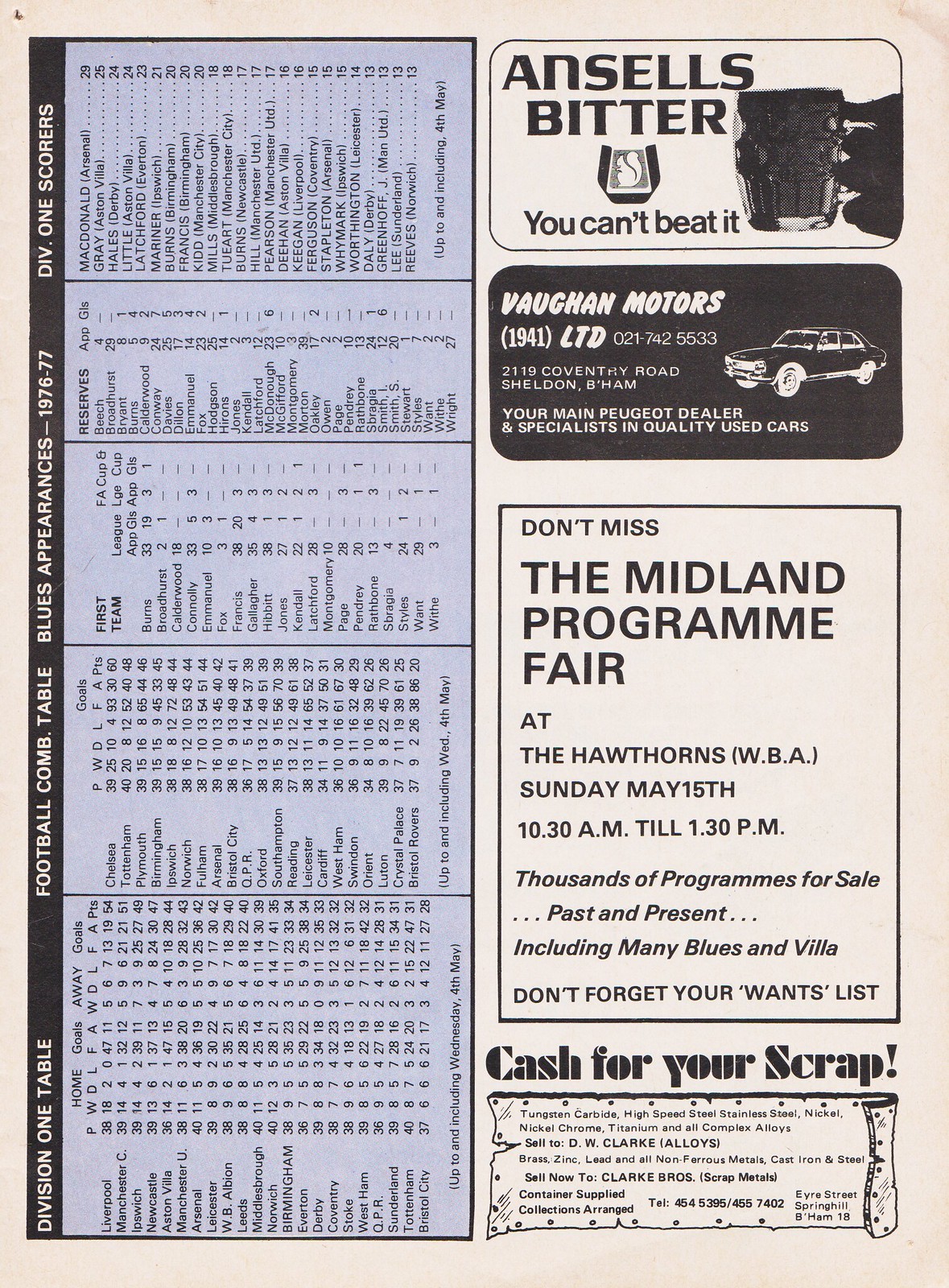This black-and-white printed page, appearing like a clipping from an old football club program, showcases a detailed snapshot of sports and advertisements from a bygone era. The page is divided into two main sections oriented in a portrait layout. The left half features a vertically formatted table, turned on its side, with a black strip header listing “Division I Table,” “Football Comb Period Table,” “Blues Appearances 1976-77,” and “Div I Scorers” in white text. Beneath these headings, detailed in small black print, are the players' names, scores, and other statistics. This side has a blue-tinted background.

The right half of the page contains four vintage advertisements stacked vertically. At the top is an ad for Ansel's Bitter, boasting "You Can't Beat It", with a logo of what appears to be a squirrel inside a cup and an adjacent image of a hand holding a glass mug. Below that is an ad for Vaughn Motors, highlighting "Vaughn Motors, 1941 Limited, Your Main Peugeot Dealer and Specialist in Quality Used Cars," alongside an illustration of a car. Next is an announcement for the "Midland Program Fair at the Hawthorne's WBA" on Sunday, May 15th, detailing timings and various program sales. The bottom ad promotes “Cash for Your Scrap,” with an image of bent scrap metal. The entire setup of the page exudes a nostalgic feel of traditional print publications, enriched with spot colors of light purple.